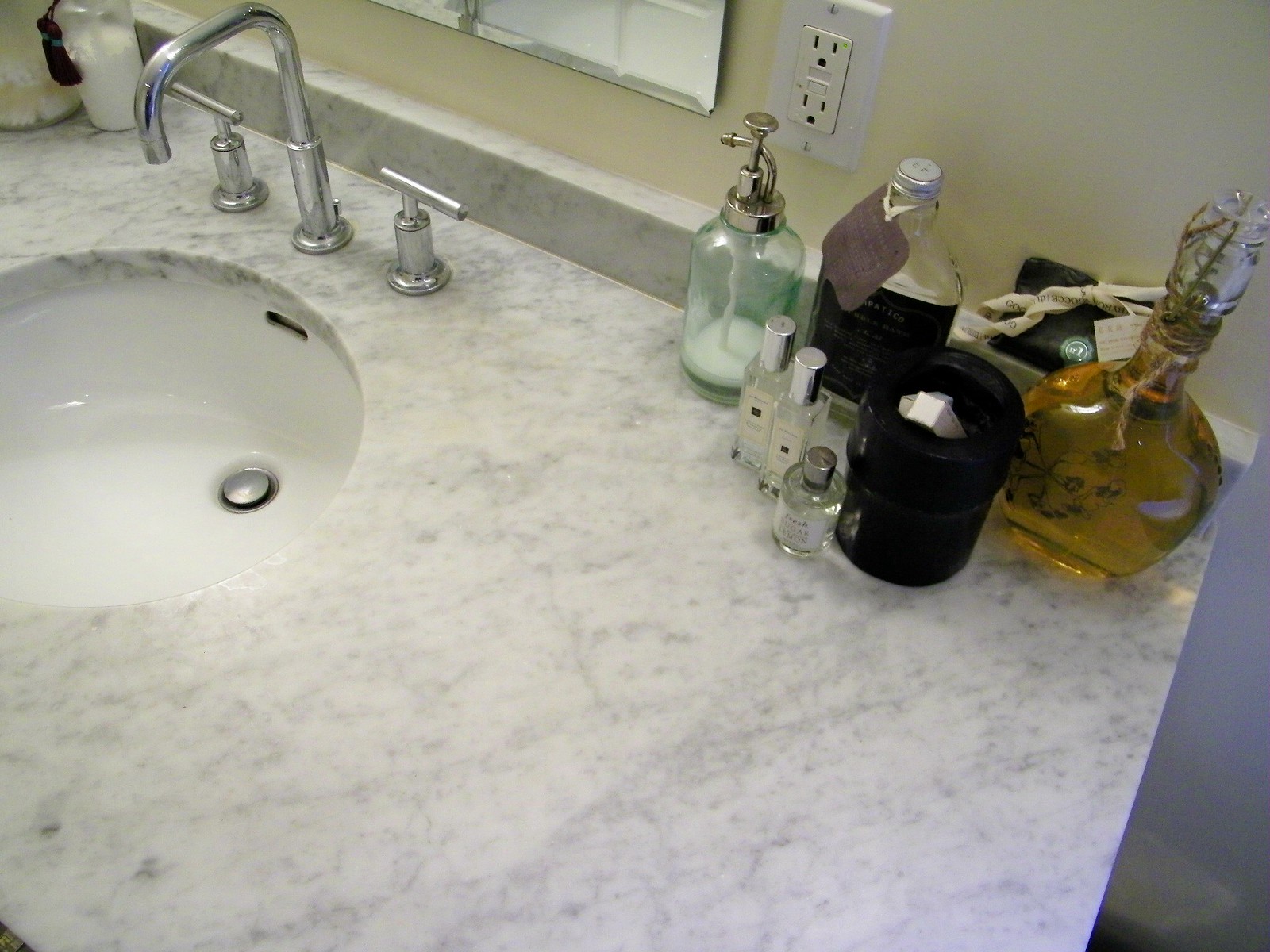A well-maintained bathroom features a pristine white marble sink, set against an off-white wall. A standard American electrical outlet is positioned on the back wall. The sink's faucet and handles have a gleaming, chrome finish. Above the sink hangs a mirror. On the left side of the sink, there are a few items: a bottle with lotion or soap, adorned with a black tassel, and a glass container filled with Q-tips. To the right, there are several glass bottles, including a collection of Jo Malone perfumes in tall, rectangular bottles, alongside a round bottle with a white label. Another decorative bottle with a white substance, presumably a large decanter of bubble bath, completes the scene.